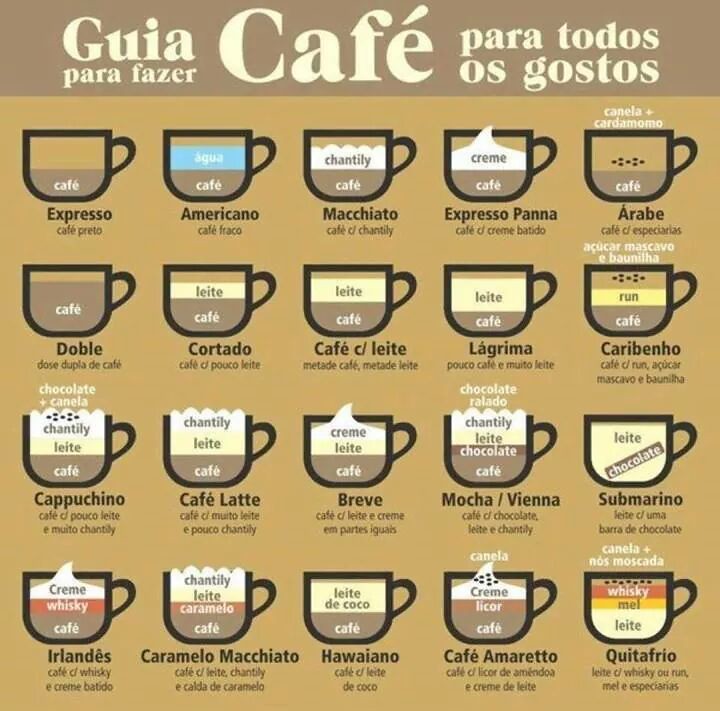This image depicts a detailed poster likely found in a coffee shop, showcasing a fascinating array of coffee varieties. The poster features a light tan background with a solid tan border across the top, where the title is adorned in creamy colored lettering. The text, seemingly in Spanish or Italian, reads "Guia Para Fazer Café Para Todos Os Gostos." Below the title, the main content is displayed on a gold background.

The layout consists of five columns and four rows, totaling 20 types of coffee, each represented by a cup outlined in black with handles facing to the right. Each cup's content is vividly illustrated with multicolored layers to indicate different ingredients. For instance, in the bottom left corner, one cup shows layers in brown (café), salmon (whiskey), and a white strip of whipped cream labeled as chantilly, demonstrating a layered coffee beverage.

Prominent coffee types include Espresso, Americano, Macchiato, Espresso Panna, and Carabinho. Unique ingredients are labeled in various colors: dark brown for café, blue for aqua, white with a ripple for chantilly, a darker yellow for rum, a lighter yellow for lychee, and red for whiskey. The poster comprehensively includes other coffees like Cortado, Café Latte, Breve, Mocha Viena, Submarino, Irlandes, Caramello Macchiato, Hawaiano, and Café Amareto, each with their respective color codes and ingredient descriptions. 

Overall, this visually appealing and informative poster serves as a perfect guide to understanding and appreciating the diverse world of coffee.